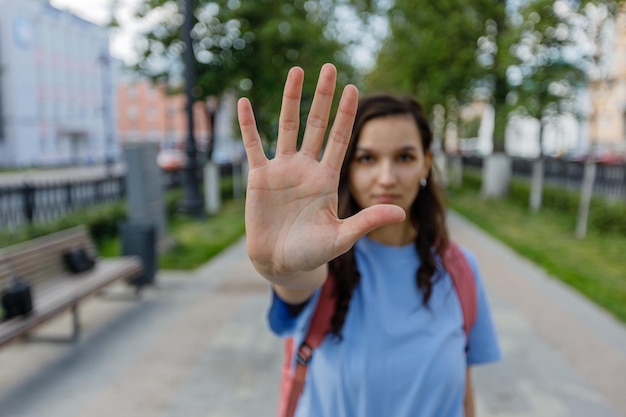In the image, a woman with long brown hair stands on a cement walkway in a park-like courtyard area. She is wearing a blue short-sleeved t-shirt and a backpack with red straps. The focus of the photograph is on her outstretched hand, which she holds up in a stop gesture, while she herself is slightly out of focus. Her expression is somber and serious, emphasizing her intent to signal someone to stop. To her left, there is a bench with what appears to be two briefcases, and a trash can beside it. The pathway is flanked by grass and lined with trees on both sides. In the background, there are buildings visible on both the left and right sides of the image, further enhancing the urban park atmosphere on what seems to be a sunny day.